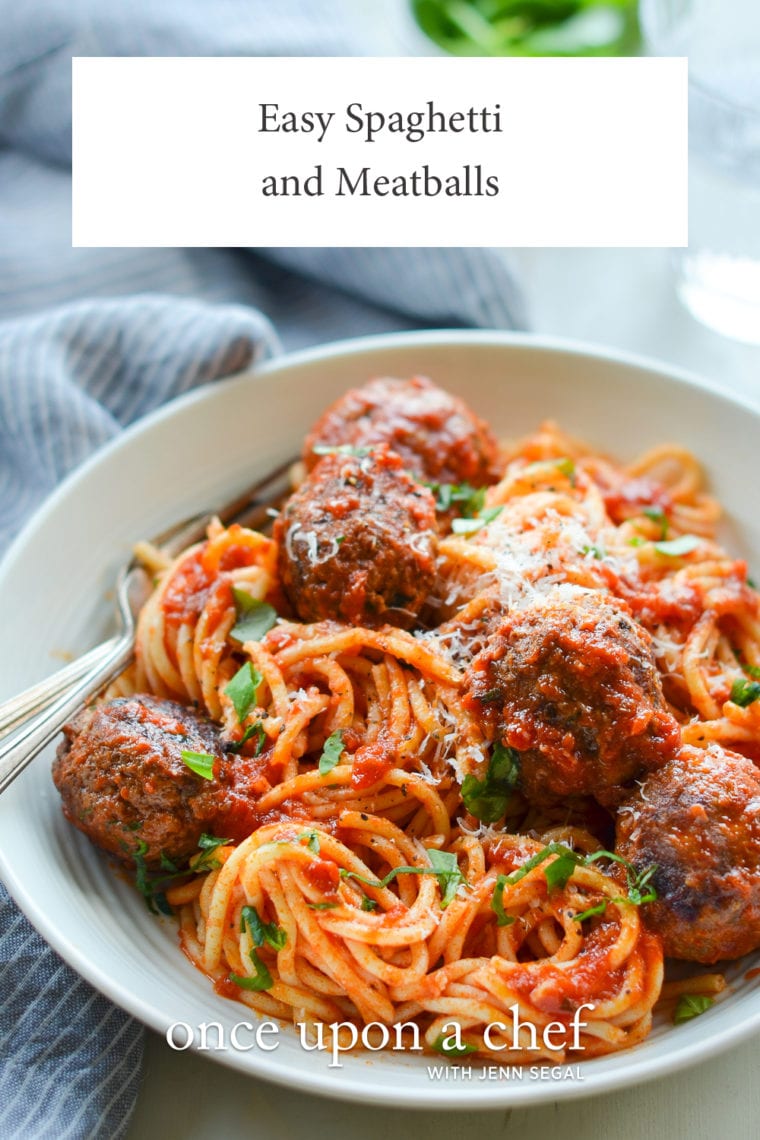The image displays a tantalizing close-up of a dish of spaghetti and meatballs, featuring a white bowl filled with glistening spaghetti drenched in rich marinara sauce and garnished with bits of basil and green parsley. Five large, juicy meatballs sit proudly atop the pasta, each lightly dusted with a tasteful sprinkle of Parmesan cheese. A silver fork rests within the dish, ready for the first bite. The plate is set against a white table, accompanied by a blue and white striped cloth, which seems to be either an oven mitt or a towel. The background is a subtle bluish-gray, enhancing the dish's vibrant colors. At the top of the image, a white text box with black lettering reads "Easy Spaghetti and Meatballs," while at the bottom, overlaid on the bowl's edge, the text "Once Upon a Chef with Jen Segal" clearly indicates the recipe’s attribution. The table also holds a few blurred objects, including a green item and an out-of-focus glass, adding depth to the composition.